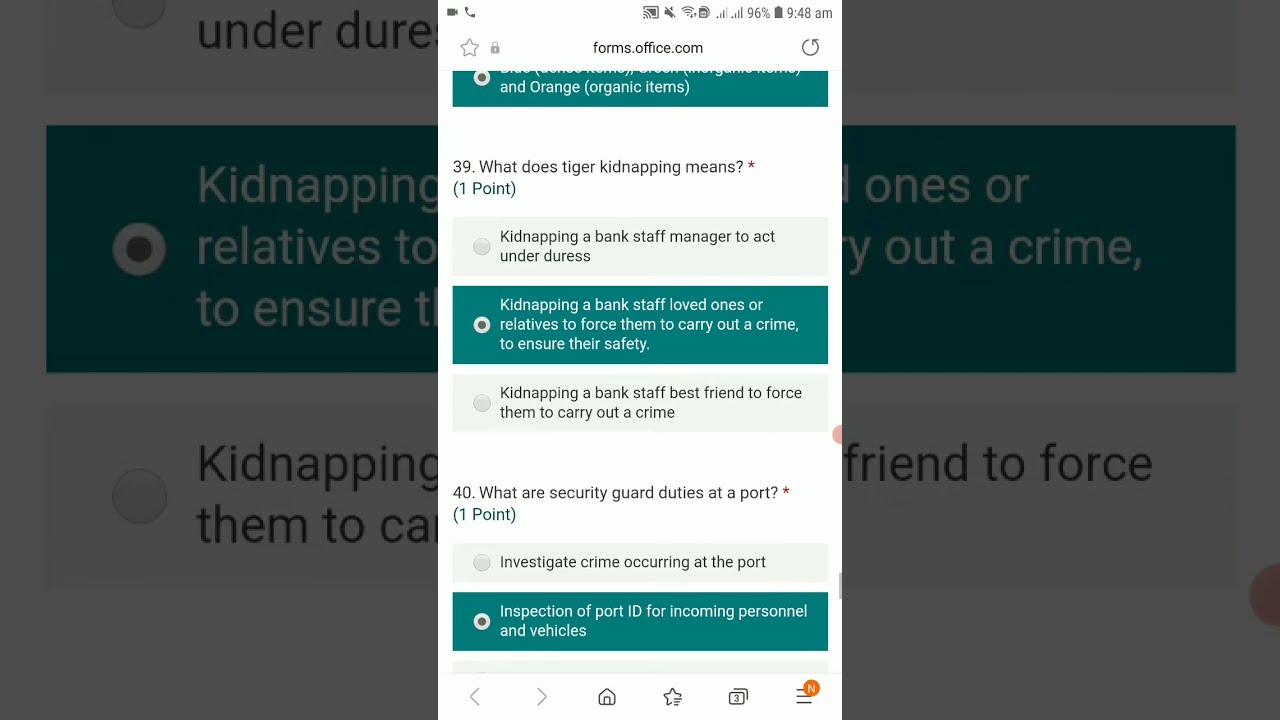This image is a screenshot of a mobile phone screen displaying a test from forms.office.com. At the top of the screen, typical phone icons are visible, including the battery level, Wi-Fi signal, and the time, which is 9:48 AM. The screen shows a blurred background that creates a border around the main content.

The main section is divided into three panels with the middle panel showing a list of questions and possible answers, with each question set against a white or green background. Question 39 asks, "What does tiger kidnapping mean?" with possible answers including: "kidnapping a bank staff manager to act under duress," "kidnapping a bank staff's loved ones or relatives to force them to carry out a crime to ensure their safety," and "kidnapping a bank staff's best friend to force them to carry out a crime." 

The selected answer for question 39 is highlighted in turquoise. Below, question 40 asks, "What are security guard duties at a port?" and includes answers such as "investigate crime occurring at the port" and "inspection of port ID for incoming personnel and vehicles," with the second answer selected in turquoise.

The left and right panels are close-ups of different sections of the main list, making it easier to read individual words but not providing the full context.

At the bottom of the screen, navigation icons such as the back button, home button, and a menu option are visible, indicating the user interface of the phone.